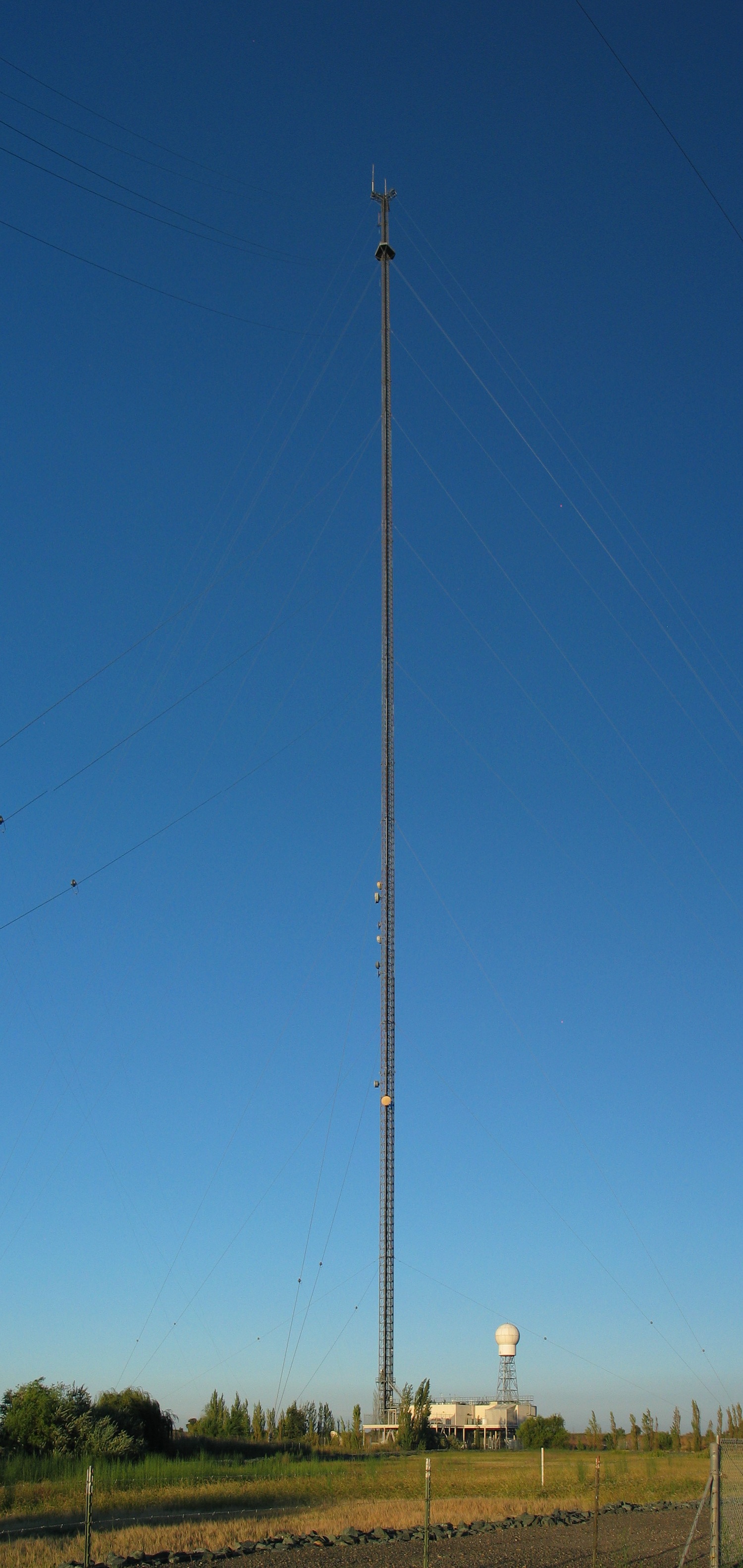This image captures a tall, gray cement pole standing several stories high against a deep blue sky. At the top of the pole, there are likely arms that could hold a couple of lights. Midway down, a disk-like structure protrudes from the pole. The sky gradually shifts to a lighter blue near the horizon, where it meets a verdant landscape. Surrounding the base of the pole are large trees and bushes to the left, and a field of grass extending across the foreground. Additionally, there is a section of fencing near the bottom of the image, with a patch of dirt visible to the right. In the distance, a water tower stands tall, completing the serene and expansive scene.